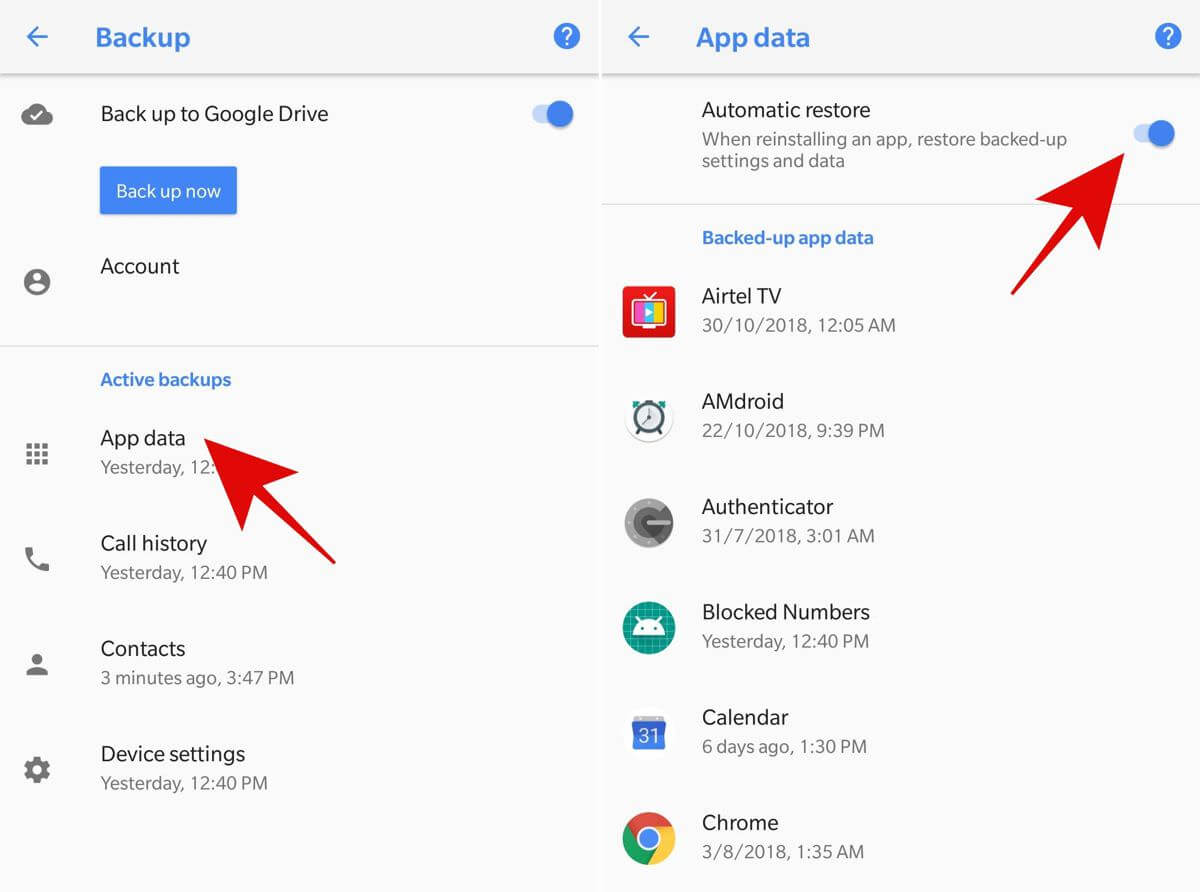This image provides a detailed guide on how to use Google Backup settings on Android devices, divided into two sections. 

The left section displays the "Backup" menu, where the "Backup to Google Drive" option is toggled on. Below this, you can see status summaries for various backup categories, such as account data, app data, and active backups. A red arrow highlights the "Active Backups" section, which includes categories like Call History, Contacts, and Device Settings.

The right section shows the "App Data" settings menu. Here, "Automatic Restore" is enabled to reinstall apps and restore backed-up settings and data. A red arrow points to this option, emphasizing how you can automatically restore data. Below are detailed timestamps for various backups:
- RTL TV: 30th October 2018 at 12:05 AM
- Android: 22nd October 2018 at 9:39 PM
- Authenticator: 31st July 2018 at 3:01 AM
- Yesterday at 12:40 PM
- Calendar: 3 days ago at 1:30 PM
- Chrome: 3rd August 2018 at 1:35 PM

Icons representing each category are displayed against a white background: Chrome with its rainbow-colored circle, Backup with a little Android robot, and RTL TV featuring a multicolored television icon.

In summary, this image serves as a detailed guide for enabling and verifying Google Backup for app data on Android devices.